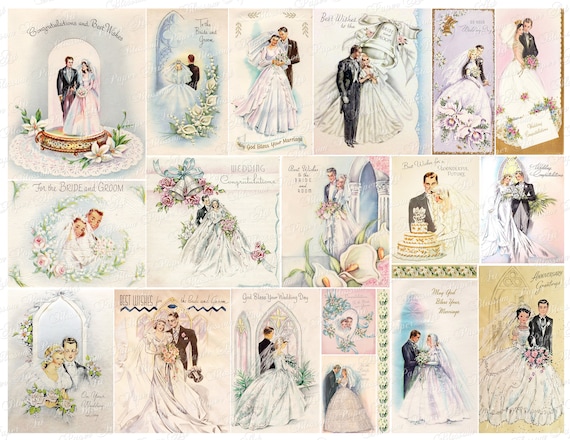This image is a meticulously curated collage of vintage wedding-themed postcards, capturing romantic scenes of brides and grooms in timeless, classic wedding attire from different eras, ranging from the 19th century to the early to mid-20th century. Each postcard features pastel illustrations, with couples depicted in various poses: dancing, holding hands, cutting wedding cakes, and gazing into each other's eyes. The brides wear long, elegant gowns with frills, lace, floral details, veils, and bouquets, showcasing the intricate fashion of the times. The grooms are in formal suits or military uniforms, suggesting a wartime context in some instances. Many cards are adorned with heartfelt messages like "Best Wishes," and framed within hearts, floral arrangements, and decorative borders. The collage layout consists of three rows: the top row with six cards, the middle with five, and the bottom with six. The detailed backgrounds range from purple and pink hues to brown, enhancing the vintage aesthetic. In some cards, additional elements like wedding bells, doors, and windows further embellish the romantic, celebratory theme. Overall, this collage beautifully encapsulates the essence of bygone wedding traditions and the enduring charm of true love.